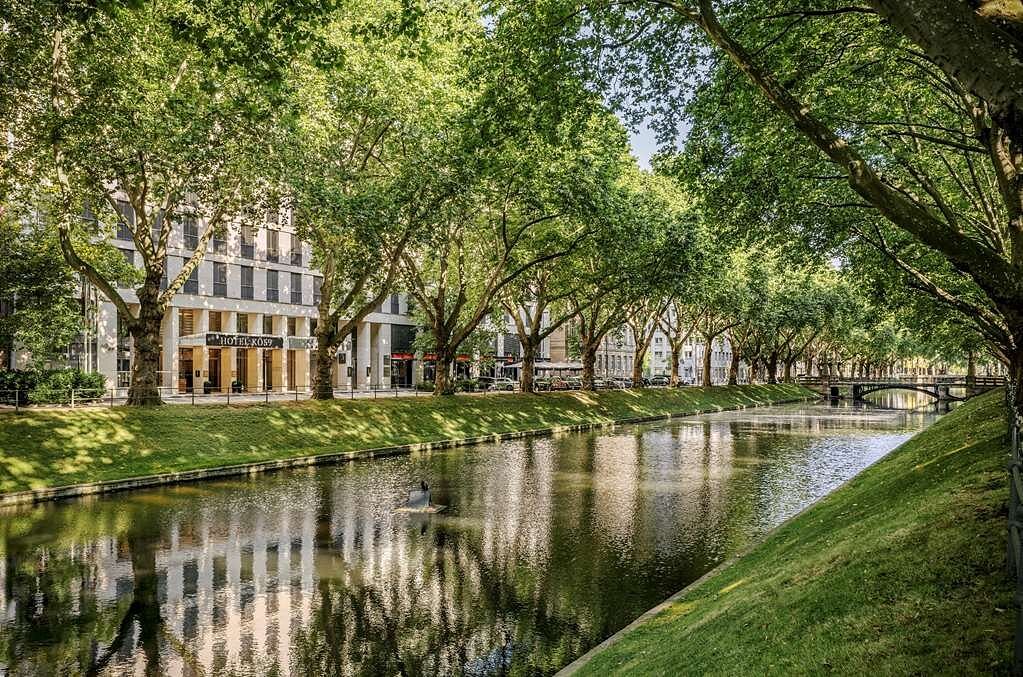The image depicts a tranquil cityscape featuring a harmonious blend of urban and natural elements, captured during the daytime. On the left side, several multi-story concrete buildings line the street, one of which has a sign reading "Hotel KO59." Beneath these buildings, there's a row of shops partially obscured by canopies with numerous cars parked in front. Central to the scene is a long, clean river or canal that runs horizontally through the image, reflecting the surrounding trees and buildings, adding to the serene atmosphere. On either riverbank, lush green grass and fully-leaved trees create a picturesque archway over the water. In the distance, there is a small footbridge crossing the river, further enhancing the scenic view. Additionally, the sky is partially visible with patches of light blue peeking through, contributing to the overall calm and beauty of the setting. This area combines natural beauty with urban infrastructure, presenting a peaceful coexistence within the city environment.